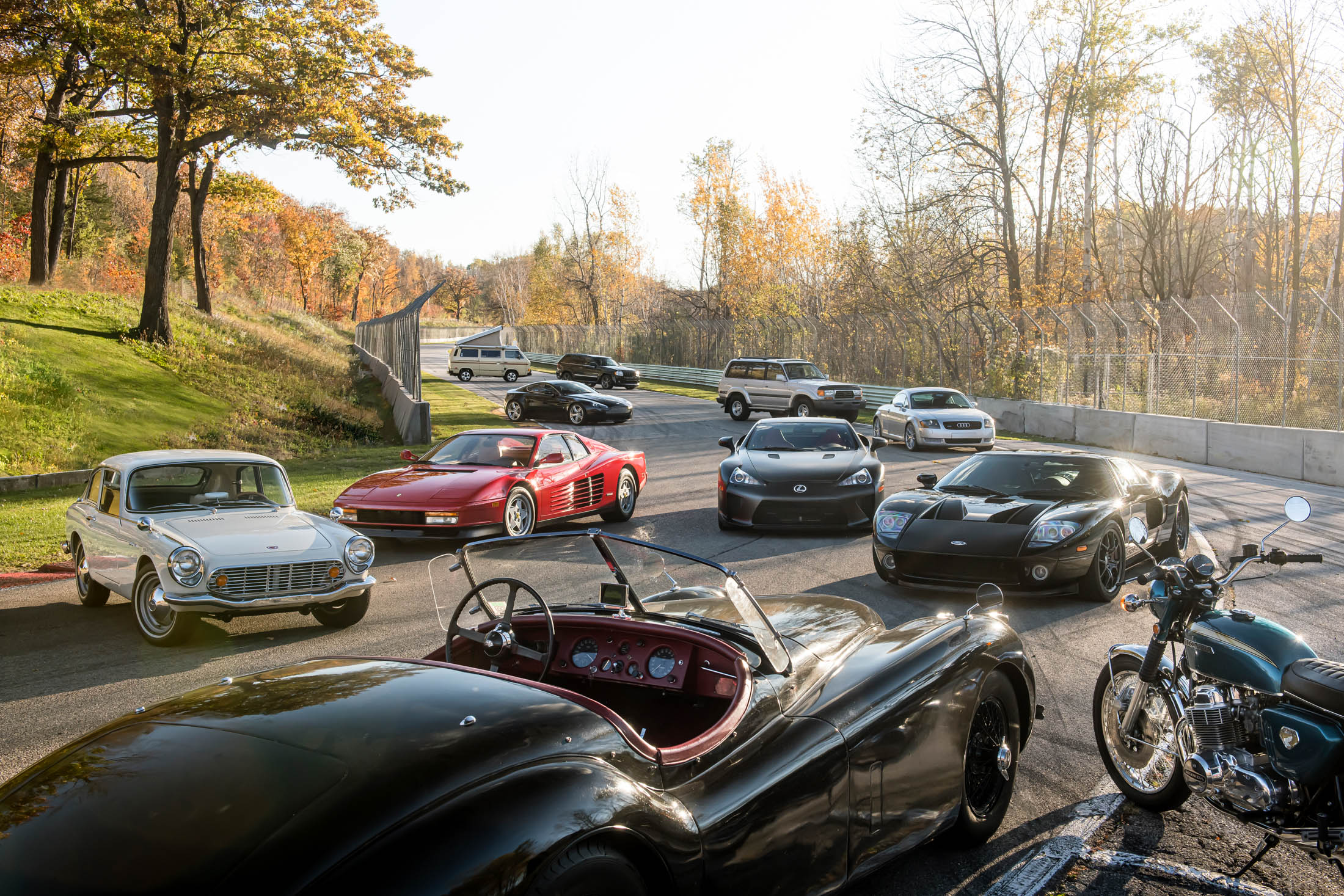The image captures an outdoor setting with a mix of fall-colored and green trees scattered in the background under a pale, almost white sky. The left side of the photo features a patch of green grass, while the remaining area is a concrete or asphalt surface populated with ten vehicles, including a motorcycle on the right-hand side. The vehicles vary widely, possibly representing iconic or generically iconic models, such as an Aston Martin reminiscent of James Bond, a red sports car akin to the General Lee, and a car hinting at KITT from Knight Rider. Notably, there’s a classic white car, a large, boat-like car resembling the Batmobile, and a blue motorcycle. The fleet includes a mix of black sports cars, a silver vehicle, a cream-colored car, a van, an SUV, and an old-fashioned station wagon in the distance. All vehicles are parked at different angles, suggesting the scene might depict a casual gathering rather than an organized event. A fence lines one side of the area, framing the eclectic assembly of cars and reinforcing the outdoor atmosphere.